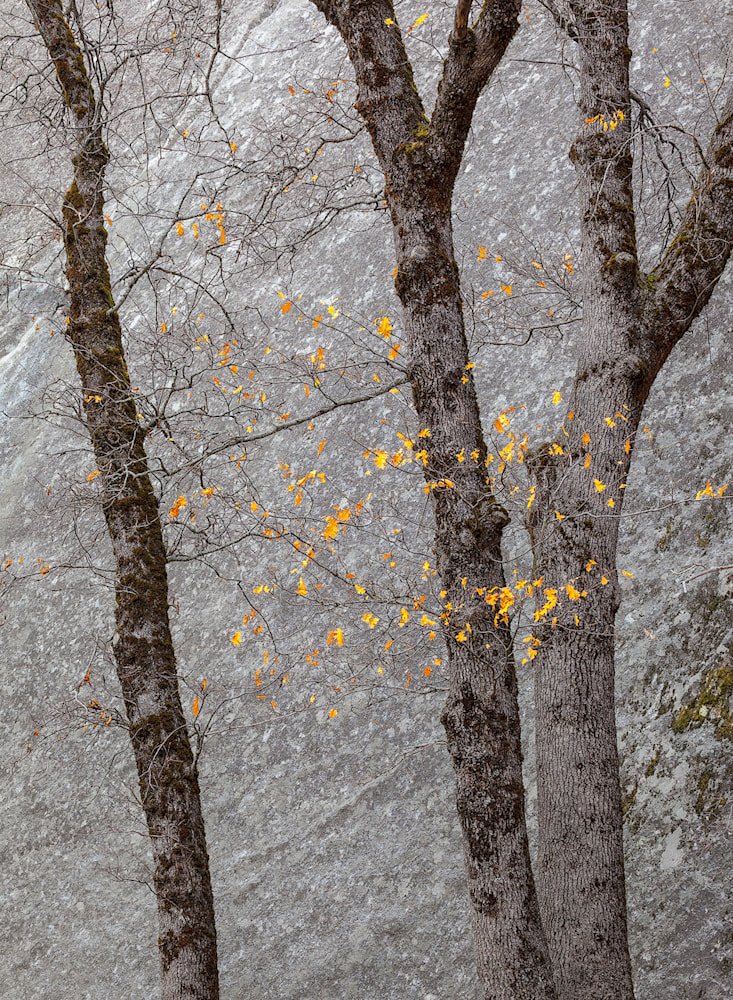This photograph captures a serene autumn scene featuring three tall, slender trees with pale bark adorned sporadically by dark gray-green moss. Their few branches are mostly leafless, aside from sparse, golden-yellow leaves clinging on as the season transitions to winter. The ground beneath the trees is bare, emphasizing their height and slender form. Behind the trees, a large, whitish-gray speckled rock face or possibly a snow drift adds a stark, wintry contrast to the scene. To the right, the edges of another tree's leaves are visible, adding a touch of complexity to the image. The overall atmosphere suggests the quietude of late fall, with the remaining leaves providing the only warmth of color against the somber backdrop.